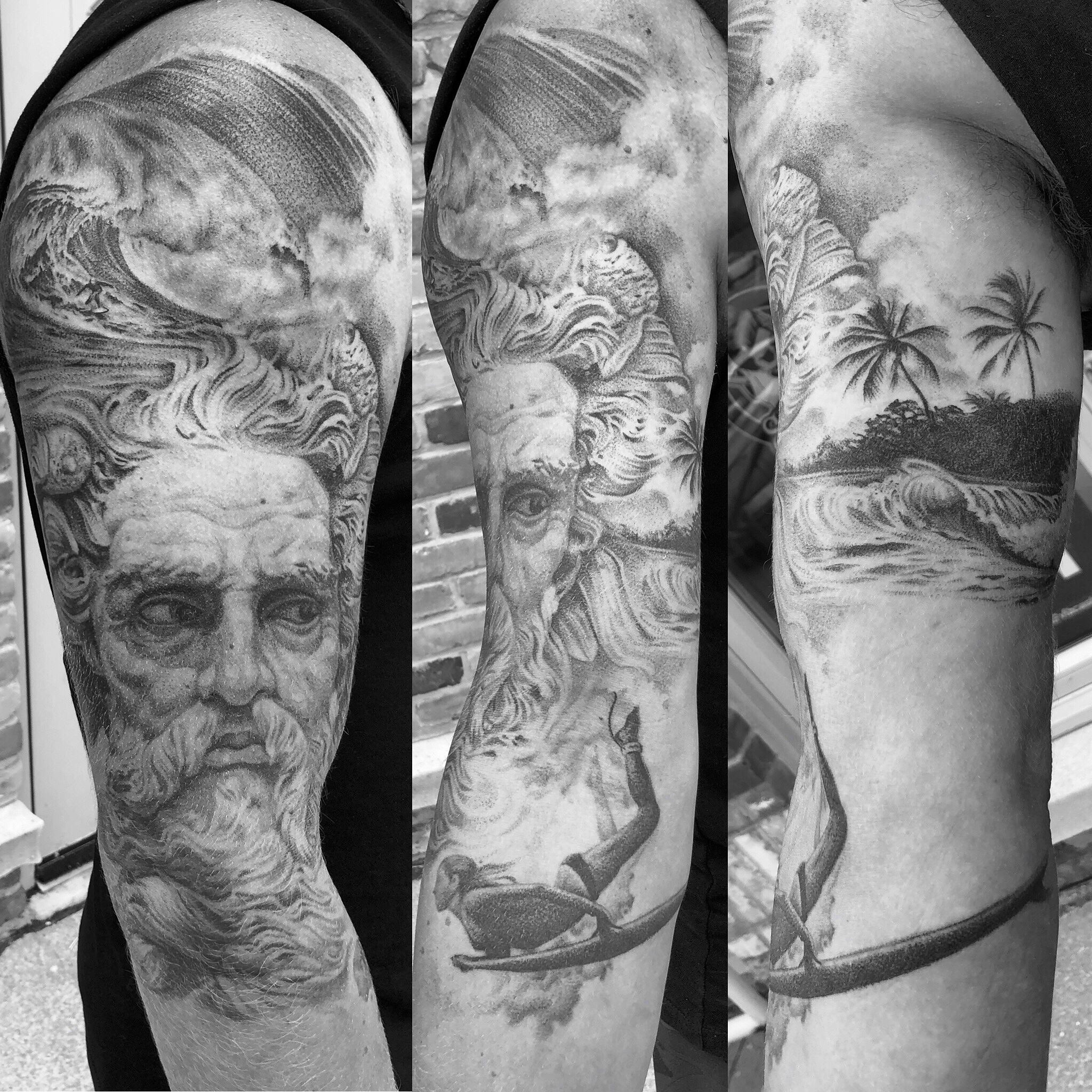This vertically oriented, black and white image is composed of three vertical panels showcasing a sophisticated full-arm tattoo. The tattoo features the intricate face of an old man, possibly resembling Zeus, with a flowing beard and hair that transforms into a dramatic ocean wave near the shoulder. The left panel highlights the man's face and the wave. The middle panel, rotating slightly towards the back of the arm, adds a detailed depiction of a woman clutching a surfboard as if diving beneath the water. Finally, the right panel reveals a picturesque beach scene with palm trees and lush foliage above the elbow, completing the continuous aquatic and natural theme that wraps around the arm.